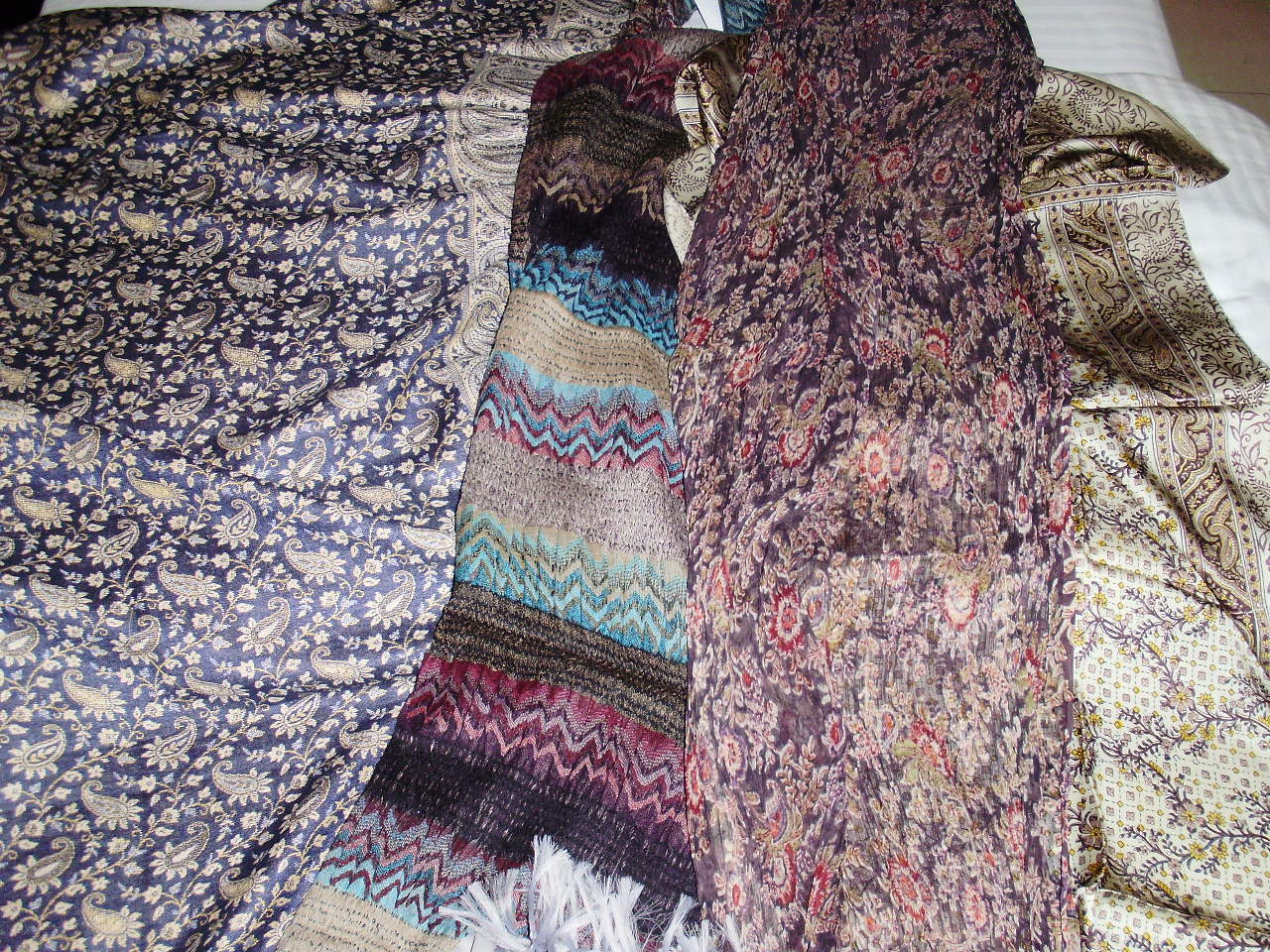The image showcases an elaborate and colorful display of beautiful, ornate scarves and fabrics, meticulously arranged on what appears to be a bed adorned with a light-colored comforter and a white satin striped sheet. Each fabric piece stands out with its intricate detailing and vibrant patterns. On the left side, there is a scarf featuring a deep magenta-purple background with cream-colored floral designs and swirl stems. Another scarf in this mix displays Native American style stitching with horizontal lines and frills at the bottom, boasting colors that range from magenta to light blue, light green, cream, browns, and blacks. Moving to the right, there are additional scarves adorned with more geometric and checkerboard patterns intertwined with beautiful interlocking rope designs. Prominently, there are fabrics with dark blue backgrounds showcasing gold paisley and botanical patterns, zigzag designs in vibrant hues of orange, yellow, tan, red, and pink, as well as a busy patterned fabric with dark black and grandmotherly floral motifs. There is also a tan fabric with yellowish geometric designs overlaid with dark brown floral patterns. Scattered within this array are more subdued pieces that resemble the elegant patterns of a pocket square. The entire composition is lively and detailed, reflecting a fusion of artistic motifs and cultural influences.